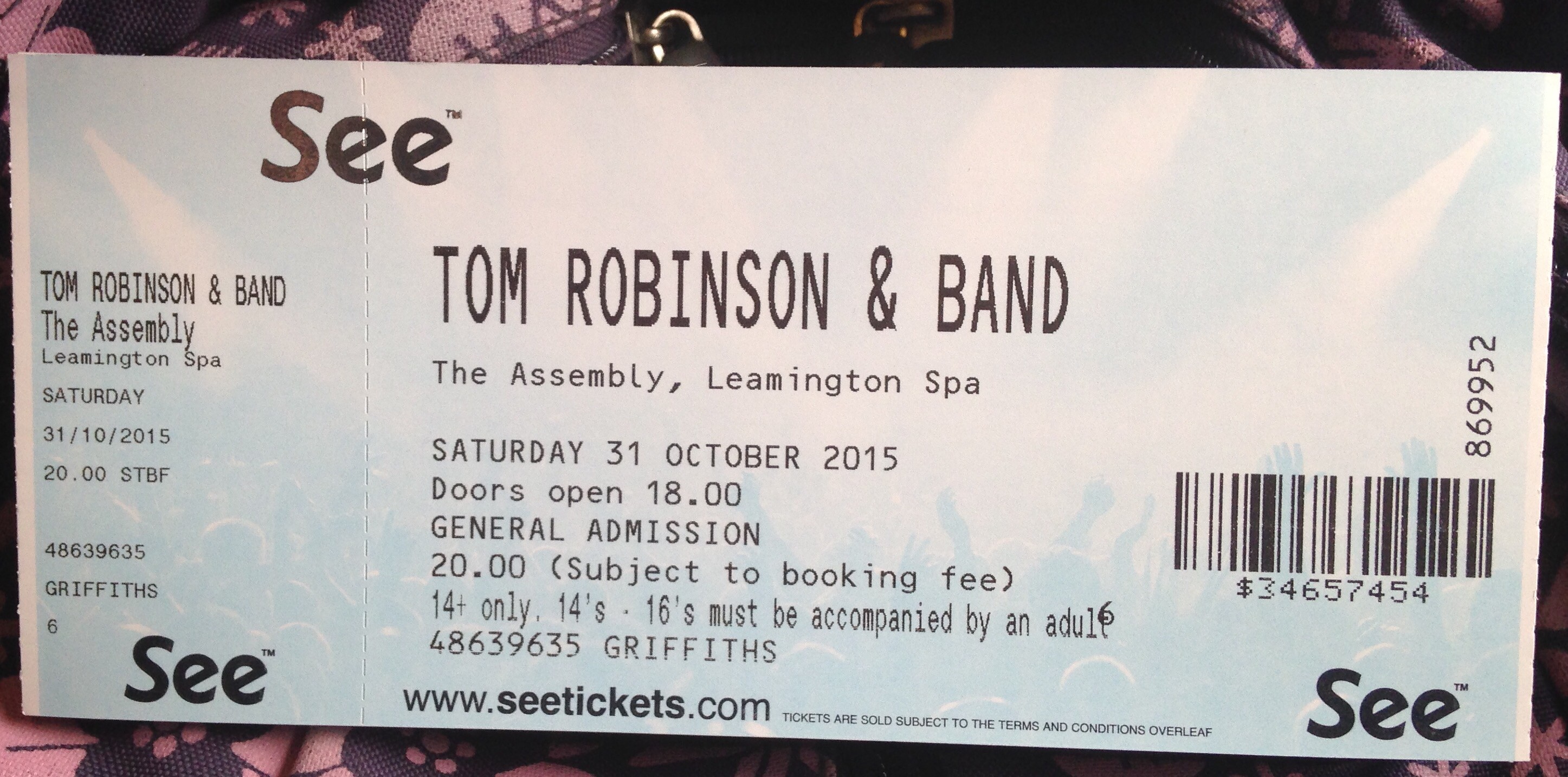This photograph showcases a detailed concert ticket for the band Tom Robinson and Band. The concert is scheduled to take place at the Assembly Leamington Spa on Saturday, the 31st of October 2015. At the top of the ticket, "see" is boldly printed, followed by the band’s name. Beneath these details, it specifies that doors will open at 18:00 (6 PM) and the general admission starts at 20:00 (8 PM), presented in military time. The ticket price is listed as $20, noting that those aged 14 to 16 must be accompanied by an adult. There is a barcode on the right for scanning upon entry and a perforated tear line on the left for the ticket stub. Additionally, the ticket mentions that it is subject to a booking fee and includes the website www.ctickets.com for further information.